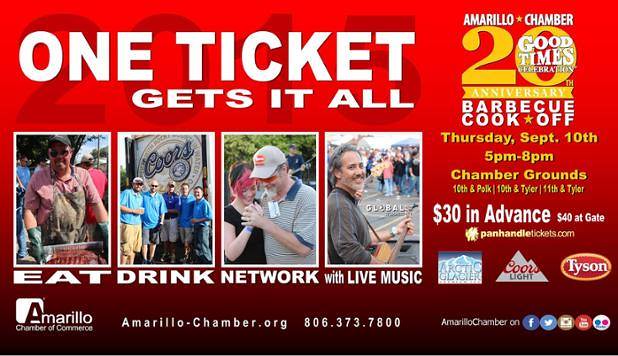This is a vibrant advertisement for a grand event hosted by the Amarillo Chamber of Commerce. The wide rectangular image features a bright red background that gradually deepens into a dark red towards the bottom. At the top left corner, atop a faint 2015 in light grayish-red, bold white text proclaims, "One Ticket Gets It All." Just beneath this are four dynamic pictures showcasing people enjoying an outdoor festival: someone grilling, friends holding drinks in front of a large Coors Alcohol sign, two people engaged in conversation, and a musician playing the guitar. Below these images, the text invites attendees to "Eat, Drink, Network with Live Music." 

In the top right corner, "Amarillo Chamber" is highlighted alongside a large golden "20" emblem and a ribbon that reads "Anniversary" in white. At the bottom, information about the "20th Anniversary Barbecue Cook-off" on Thursday, September 10th, from 5 p.m. to 8 p.m. at the Chamber Grounds (10th and Polk, 10th and Tyler, and 11th and Tyler) is detailed. Tickets are $30 in advance and $40 at the gate, available on panhandletickets.com. The event is sponsored by Arctic Glacier, Coors Light, and Tyson. The advertisement concludes with contact details: AmarilloChamber.org and phone number 806.373.7800.